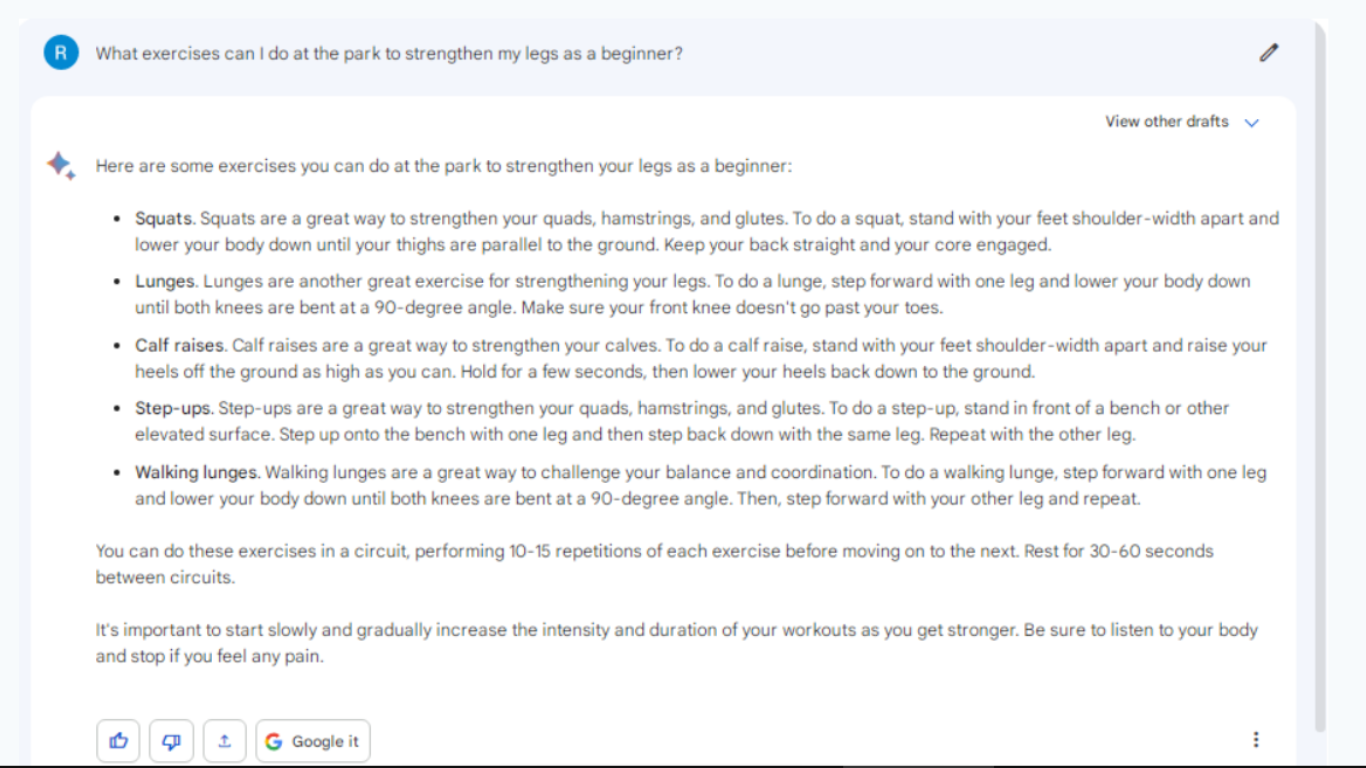The image features a question-and-answer format, aimed at providing guidance on beginner leg-strengthening exercises that can be performed in a park. The top section displays a blue circular logo with a white "R" in the center. 

The question posed is: "What exercises can I do at the park to strengthen my legs as a beginner?"

The answer is detailed and includes the following exercises with instructions:

1. **Squats**: 
   - Description: Squats are effective for strengthening the quads, hamstrings, and glutes.
   - Instructions: Stand with feet shoulder-width apart, lower your body until thighs are parallel to the ground, keeping your back straight and core engaged.

2. **Lunges**:
   - Description: Lunges are excellent for leg strength.
   - Instructions: Step forward with one leg and lower your body until both knees are bent at a 90-degree angle. Ensure your front knee does not extend past your toes.

3. **Calf Raises**:
   - Description: Calf raises focus on strengthening the calves.
   - Instructions: Stand with feet shoulder-width apart, raise your heels as high as possible, hold for a few seconds, then lower your heels back to the ground.

4. **Step-Ups**:
   - Description: Step-ups are great for targeting the quads, hamstrings, and glutes.
   - Instructions: Stand before a bench or elevated surface. Step up with one leg, then step back down with the same leg. Repeat with the other leg.

5. **Walking Lunges**:
   - Description: Walking lunges challenge balance and coordination.
   - Instructions: Step forward with one leg and lower your body until both knees are bent at a 90-degree angle. Step forward with the other leg and repeat.

Additional advice mentions performing these exercises in a circuit, with 10 to 15 repetitions each before moving on to the next exercise. It recommends resting for 30 to 60 seconds between circuits and advises starting slowly, gradually increasing the intensity and duration of the workout. It emphasizes the importance of listening to your body and stopping if any pain is felt.

At the bottom of the image, there are icons for liking or disliking the content (thumbs up or thumbs down), downloading it, and using a "Google it" button for further information.